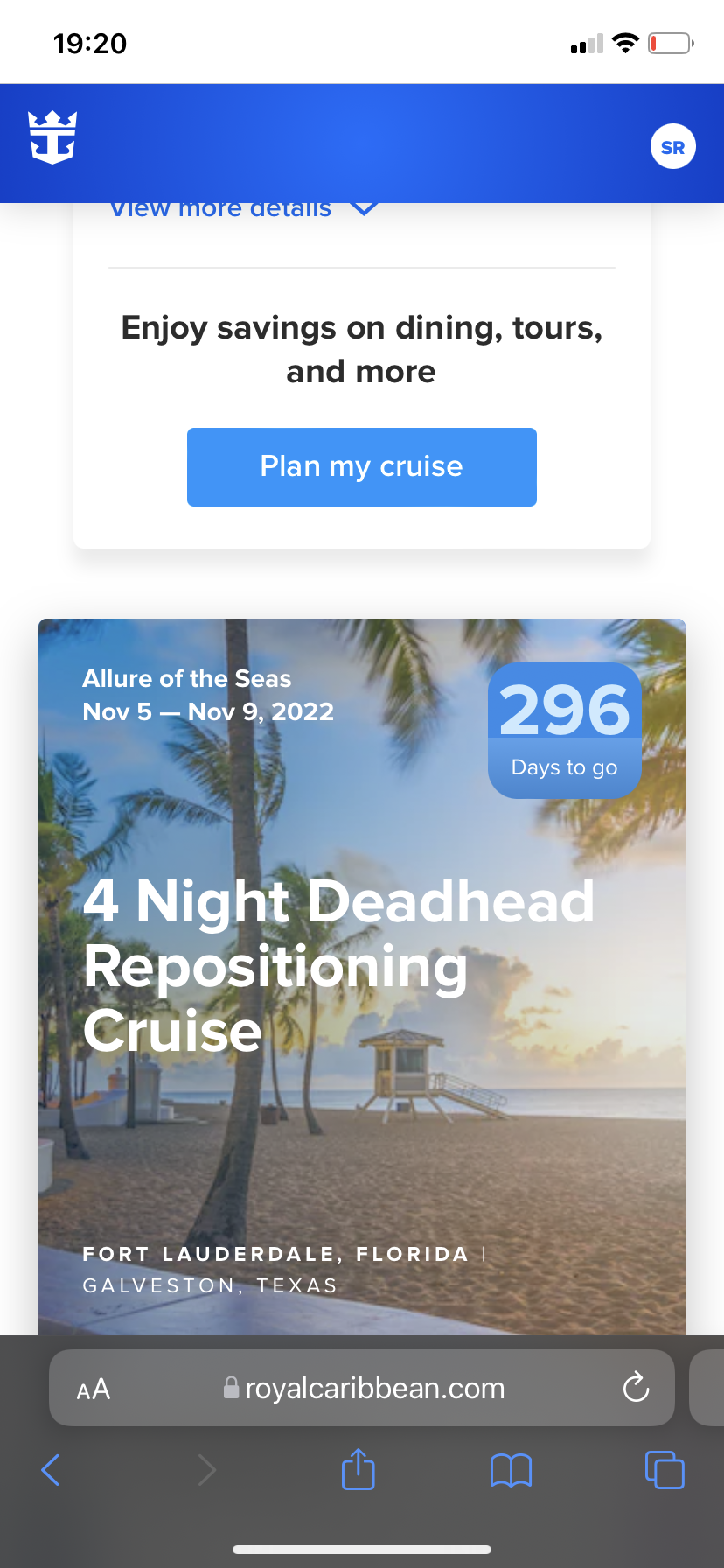A screenshot captures a user browsing the Royal Caribbean website on Safari browser in dark mode on their iPhone. At the top of the homepage, framed by a blue band, is the Royal Caribbean logo—a clever crown-anchor hybrid. The user, signed in as 'SR,' has scrolled down to a promotional section that offers savings on dining, tours, and more. A prominent blue button invites them to "Plan My Cruise." Further down, details of an upcoming cruise are displayed: the Allure of the Seas, set to sail from November 5th to 9th, 2022, with 296 days remaining. This four-night deadhead repositioning cruise will travel from Fort Lauderdale, Florida to Galveston, Texas. Accompanying this itinerary is a stunning image of a luxurious beach at sunset, palm trees swaying gently—likely illustrating one of the serene stops on the cruise.